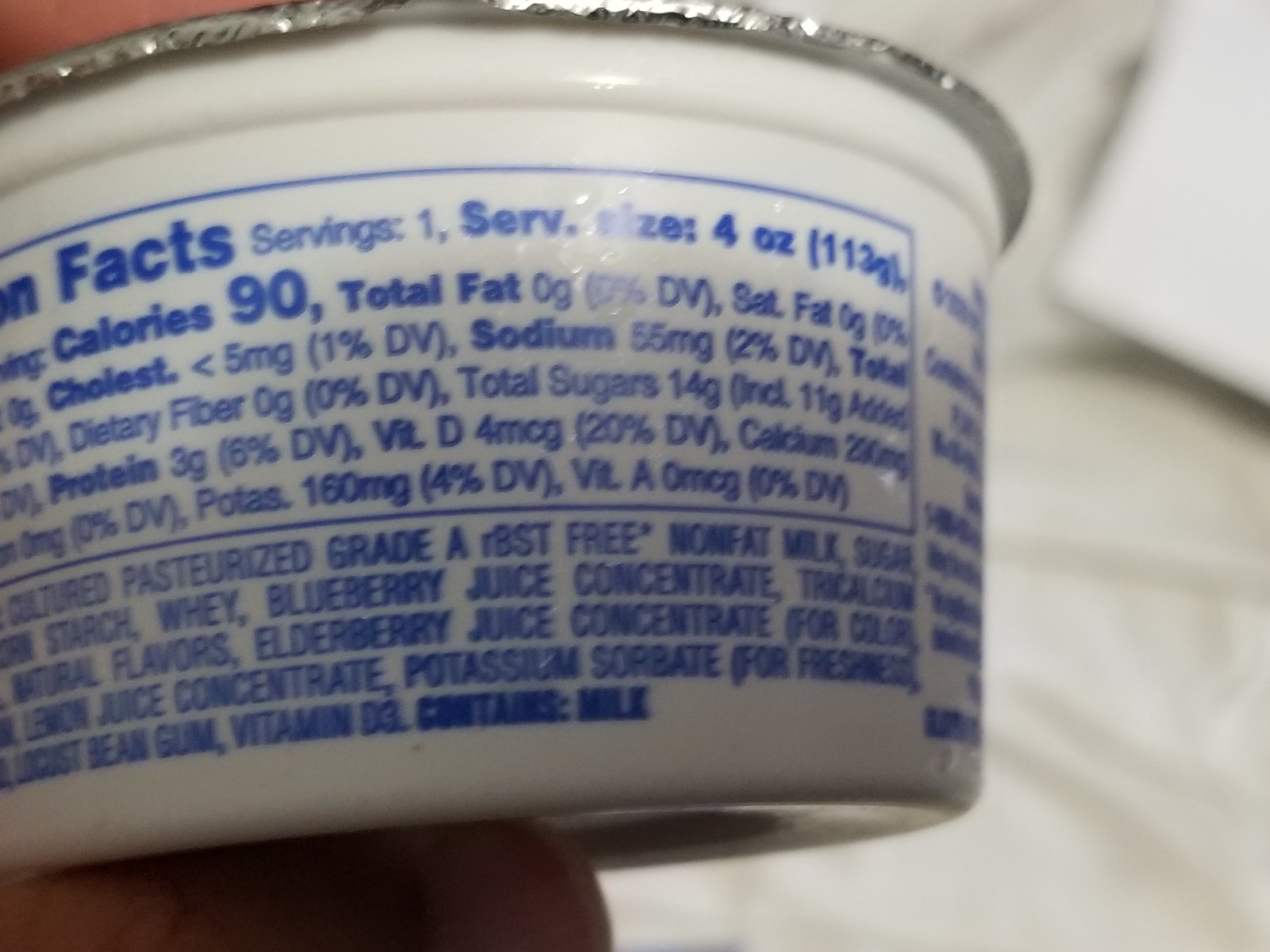Close-up image of a white plastic container featuring nutritional and ingredient information in medium blue text. The container is sealed with an unopened foil lid, and a thumb is visible underneath, holding it up. The background appears to be white. The text on the container reads:

Nutrition Facts per Serving:  
- Serving Size: 4 ounces  
- Calories: 90  
- Total Fat: 0g  
- Saturated Fat: 0g  

Ingredients:  
- Cultured, pasteurized, Grade A, RBST-free nonfat milk  
- Sugar  
- Cornstarch  
- Whey  
- Blueberry juice concentrate  
- (illegible)  
- Natural flavors  
- Elderberry juice concentrate (for color)  
- Lemon juice concentrate  
- Potassium sorbate (for freshness)  
- (illegible) bean gum  
- Vitamin D3  

Contains: Milk